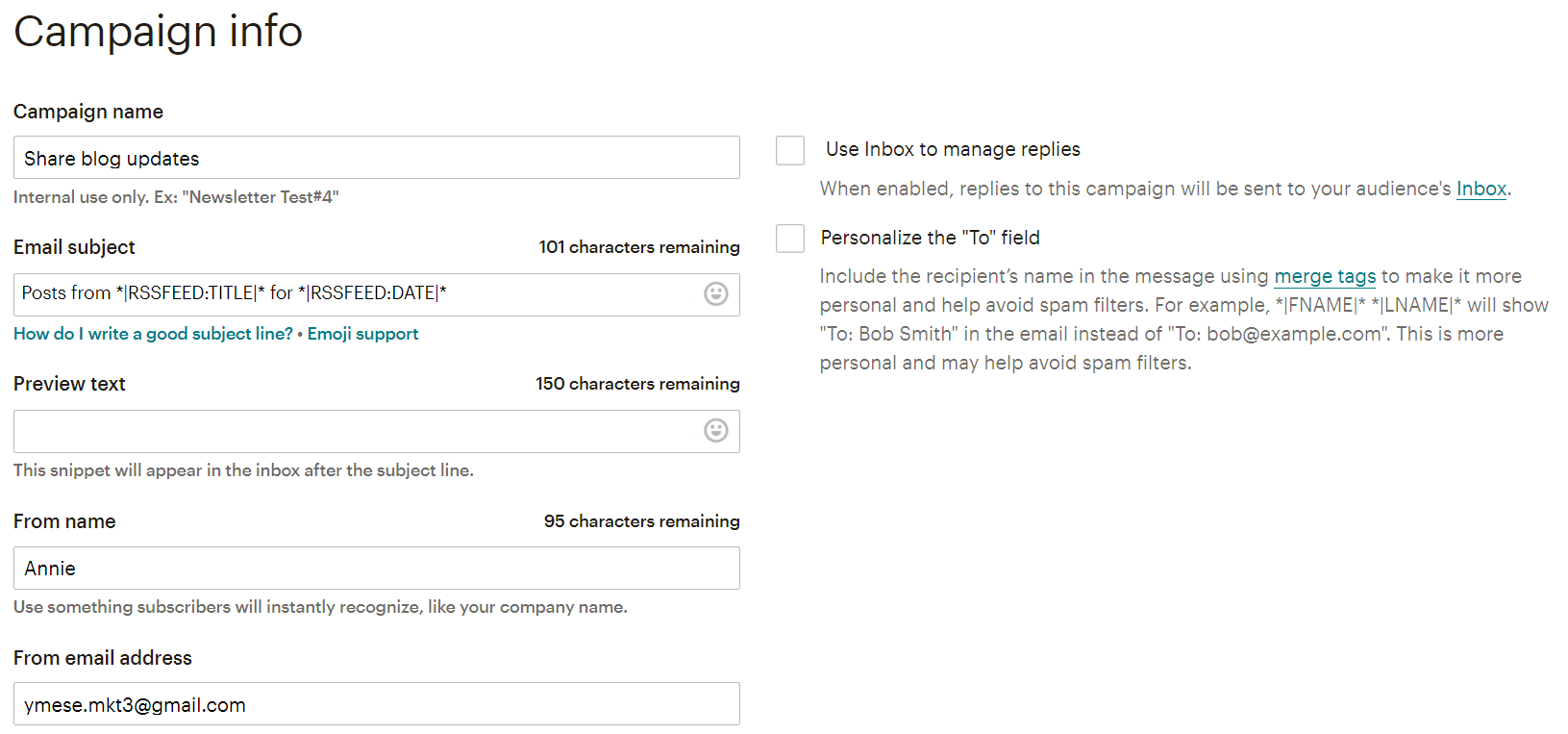On the upper left corner of the image, there is campaign information displayed against a white background. Below this section, "Campaign Name" is labeled on the left, and its data field reads "Share Blog Updates." The text "Internal Use Only" is situated below it with an example labeled "EX newsletter test number four."

Further down, there is a section labeled "Email Subject" with a note indicating 101 characters remaining. In the data field, it reads "Post from *|RSS:FEED:TITLE|* for *|RSS:FEED:DATE|*." Beneath this, in blue text, it states "How do I write a good subject line?" followed by "Emoji Support."

The subsequent section is labeled "Preview Text" with 150 characters remaining, and the data field for this section is empty. A note explains that this snippet will appear in the inbox after the subject line.

Next, the "From Name" field has 95 characters remaining and the name "Annie" (spelled A-N-N-I-E) is entered. It's advised to use something that subscribers will instantly recognize, like the company name. The "From Email Address" field contains "ymese.mkt3@gmail.com."

On the right side of the image, there is an option to "Use Inbox to Manage Replies," with a description indicating that when enabled, replies to this campaign will be sent to the audience's inbox. There is a checkbox for this option, which is currently unchecked.

Finally, at the bottom, there is a prompt labeled "Next," followed by the instruction to "Personalize the To Field."